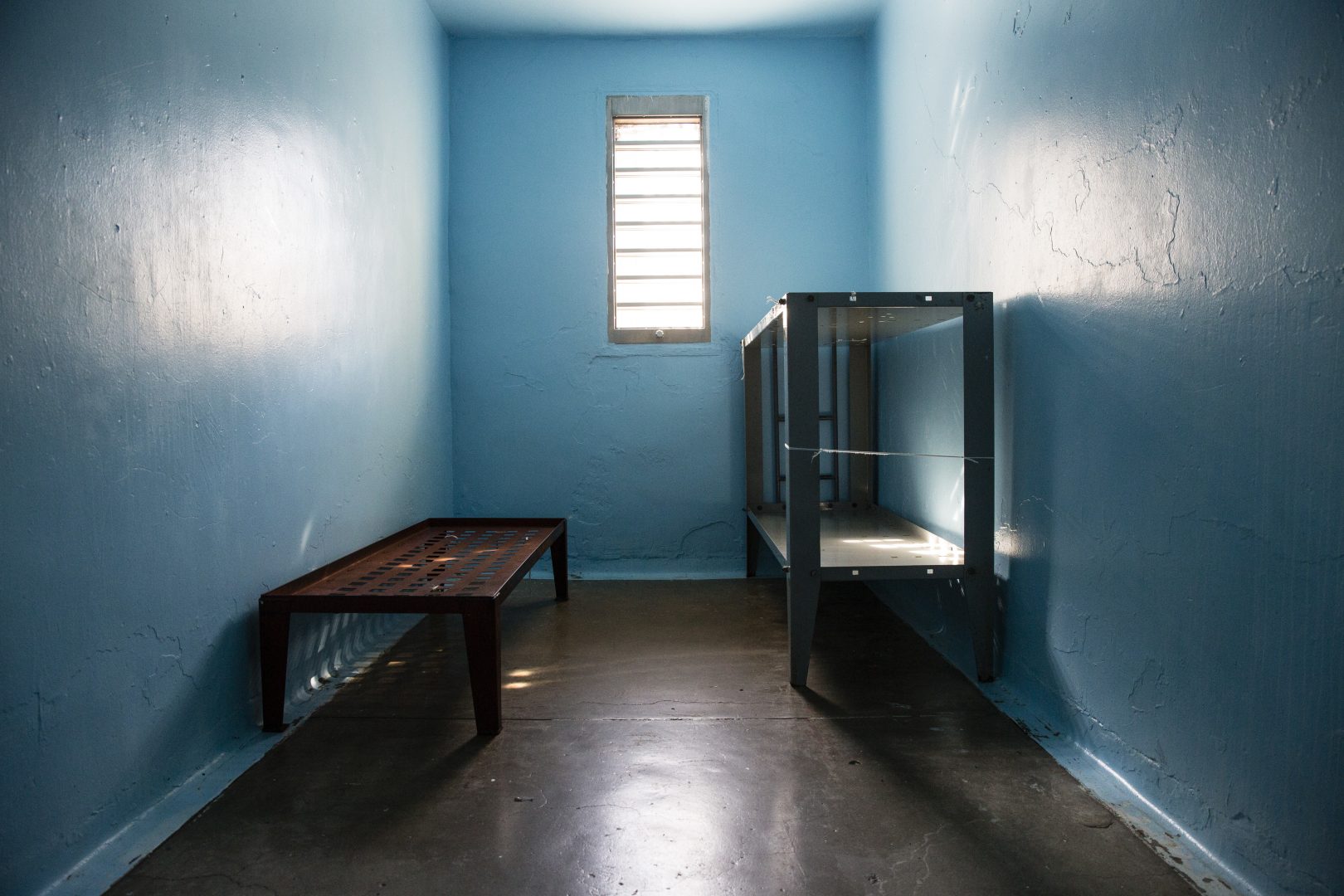The image depicts a stark, empty jail cell featuring sky-blue walls and a dark brown industrial linoleum floor. Nestled in the back wall, a narrow, portrait-shaped window with horizontal grill work allows bright morning sunlight to spill into the room, casting shadows on the ceiling and walls. The room’s interior is sparsely furnished with a rudimentary, low-level, dark wooden bench on the left side, and a gray metal structure resembling a set of bunk beds, devoid of mattresses, positioned on the right. The gray floor appears concrete-like, and the blue walls show signs of chipping and indentations, adding to the cell's austere and neglected atmosphere.